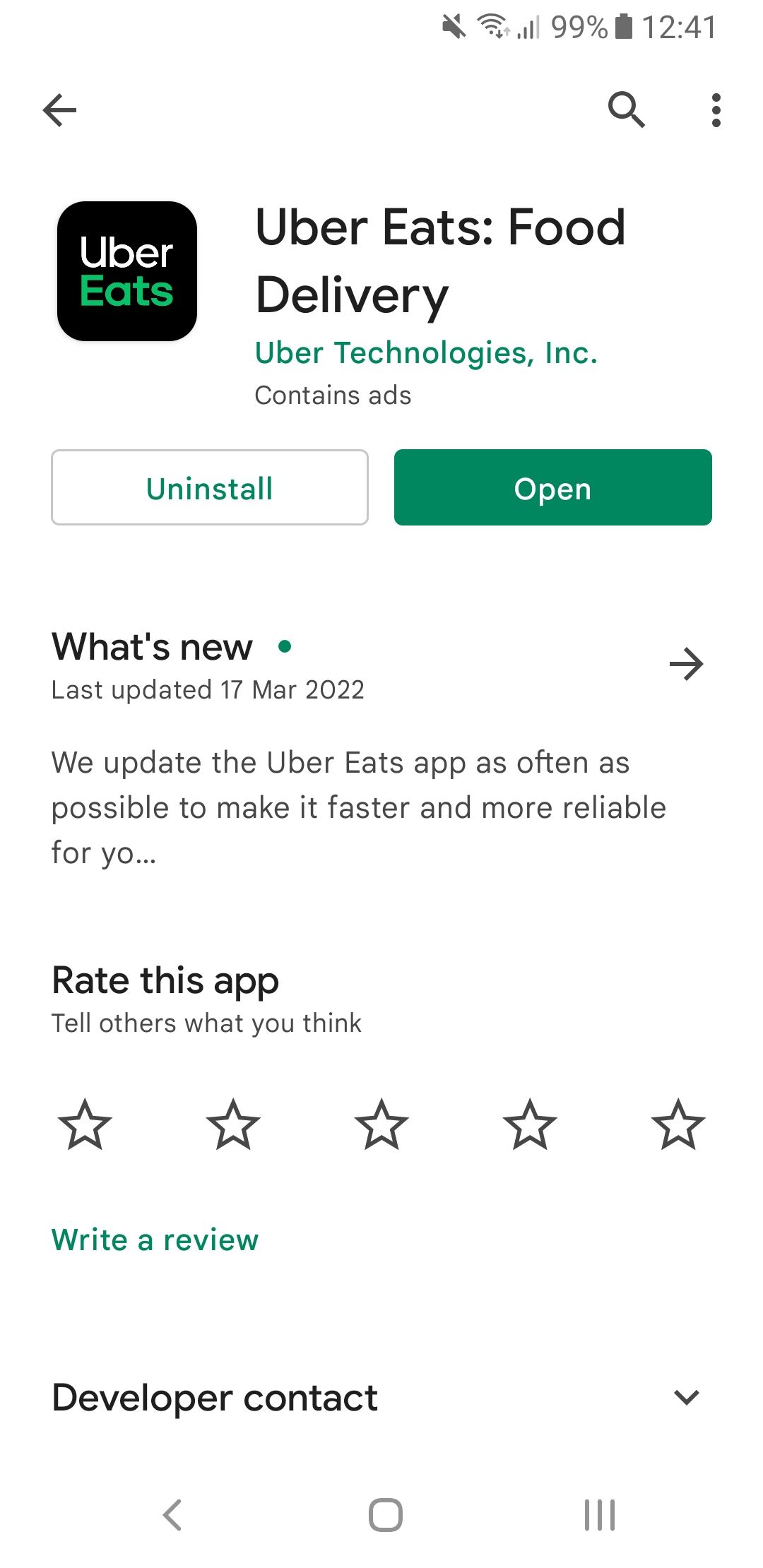This screenshot depicts the Uber Eats app page as shown on a smartphone. The background is predominantly white, with the iconic Uber Eats logo prominently displayed on the upper left. The logo features "Uber" in black lettering and "Eats" in green. To the right of the logo, the title "Uber Eats: Food Delivery" is written in black letters, followed by the app developer’s name, "Uber Technologies Inc." in green lettering, and a note saying "Contains ads" in grey.

This page is from the app store section of the phone where users can manage their apps. It's clear that the Uber Eats app is already installed on the device, as indicated by the presence of two buttons: "Uninstall" and "Open."

Below these buttons, there's a section titled "What’s New," highlighting the latest update, which was on 17 March 2022. A brief message states, "We eat, we update the Uber Eats app as often as possible." Moving further down, users are prompted to rate the app, with five stars shown underneath the text "Rate this app." Additionally, there's a green button labeled "Write a review."

At the bottom of the screen, basic navigation buttons are visible, which are typical on most smartphones. This detailed screenshot provides a clear overview of the Uber Eats app's management interface on a mobile device.